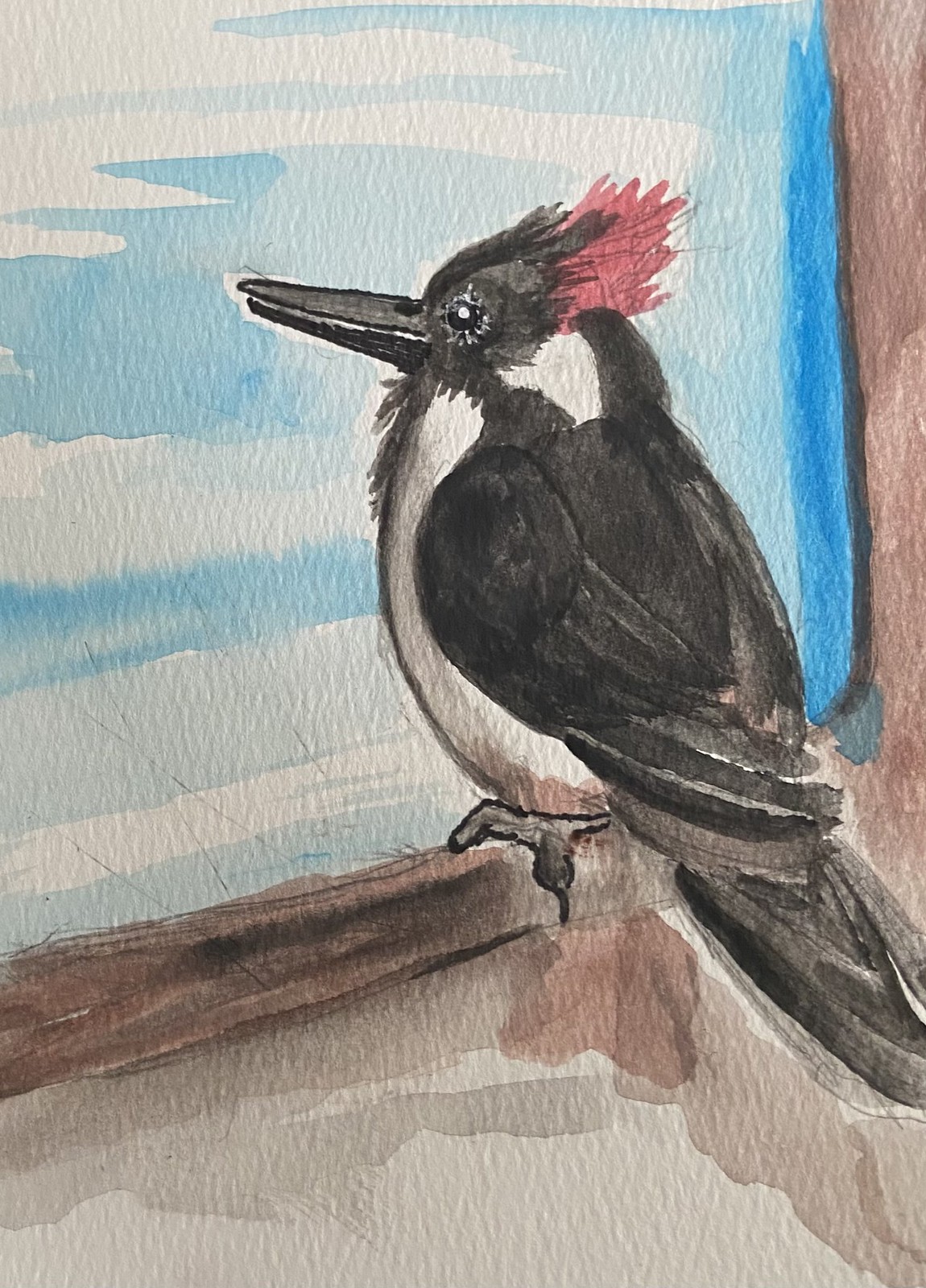This detailed watercolor painting depicts a bird resembling a woodpecker perched on a piece of wood, potentially driftwood or a tree branch. The background features shades of blue, rendered lightly to give an impressionistic feel. The wood is painted in a brown hue, with smooth bark on the main trunk transitioning to a darker shade at the jutting branch. The bird has striking black and white plumage: its back, wings, and face are black, while its chest and belly are white. Notably, it has a red crest on its head and a white spot behind its black eyes. The bird's long, pointed beak and claws are both black, adding to its distinctive appearance.